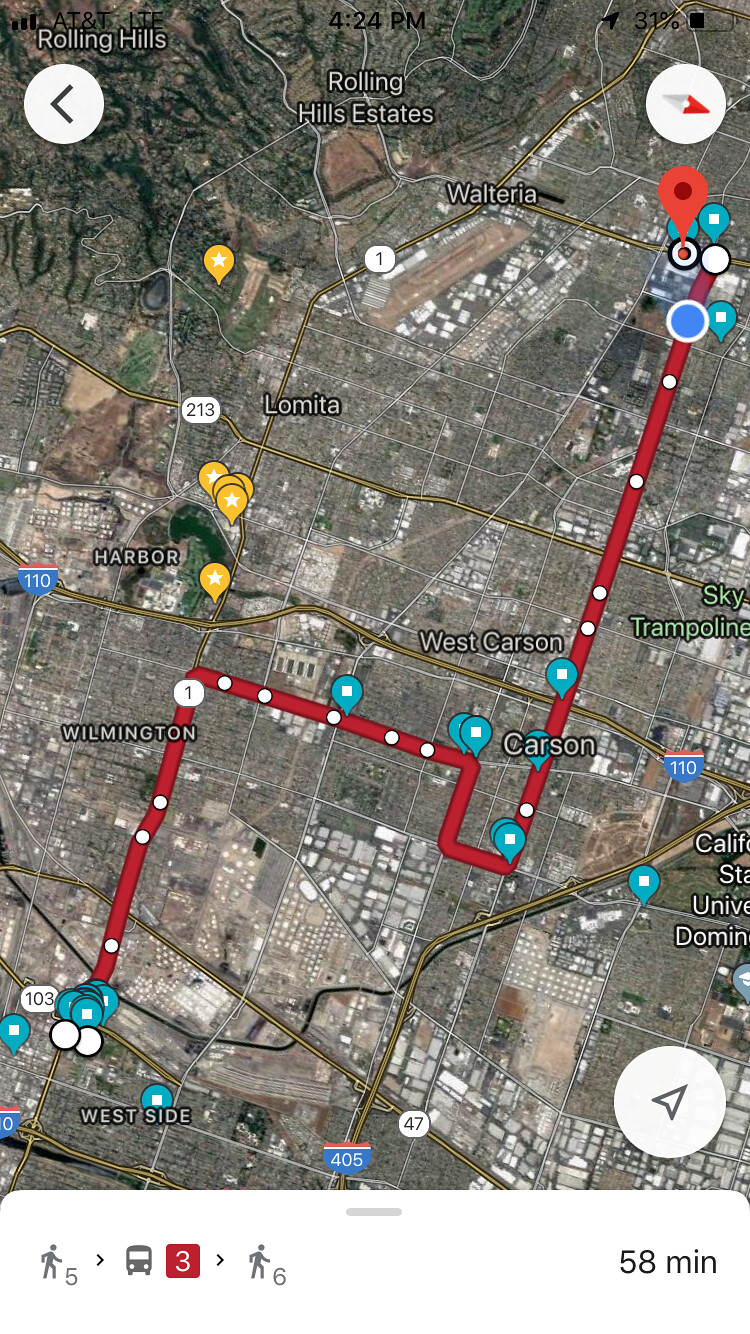Screenshot of a navigational map:

This detailed screenshot of a map shows a route highlighted in red with various blue teardrop markers denoting stops along the path. At the bottom right, it indicates a total travel time of 58 minutes. The bottom left features three icons: a person with the number 5 beside it, a bus symbol with the number 3 surrounded by a red outline, and another person with a number 6 next to it. The map is crisscrossed by several streets and highways, with prominent yellow paths representing highways or freeways. Notable highways on the map include "Row 5" marked in blue with a red top, and "110". Some of the white-bubbled highway designations read "1", "47", "213", and "103".

Text elements at the top of the screen include "AT&T," "ITE," "4:24 PM," and a battery indicator showing "31%." Specific locations labeled on the map include "Rolling Hills" at the top left, "Rolling Hills Estates" at the center top, and other areas like "Walteria," "Lomita," "West Carson," "Sky Trampoline," "Carson," "Wilmington," and "Westside." The map serves both as a geographic guide and a real-time navigation aid, as inferred from its layout and the digital information displayed.